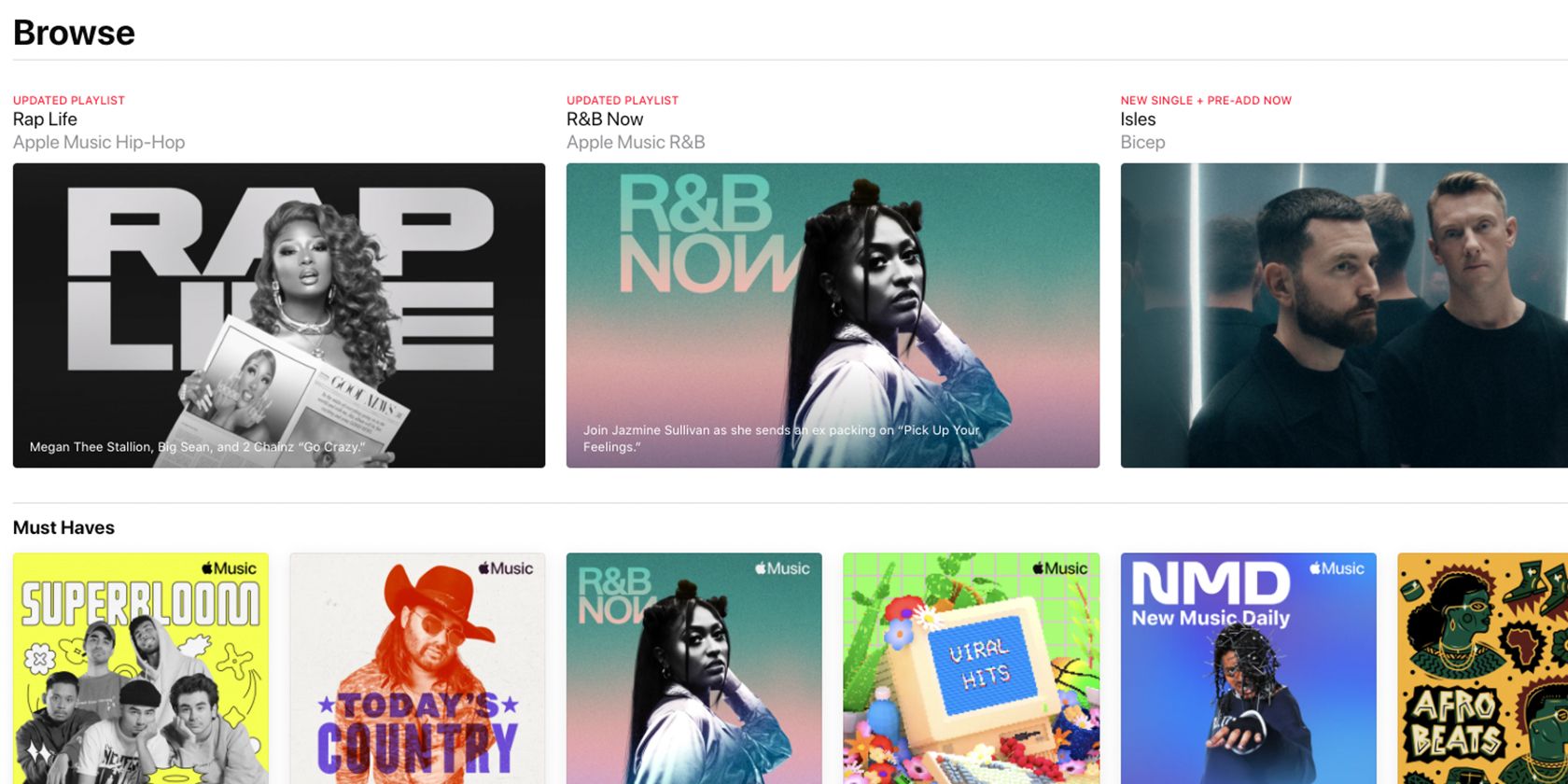The image displays an Apple Music menu showcasing a variety of songs and records from different artists. At the top, in bold black letters, it says "Browse." A horizontal line extends across the width of the image just below the title.

Directly underneath, there are three prominent album covers or record pictures featuring different artists. The first one highlights the "Rap Life" playlist under Apple Music Hip-Hop, featuring Megan Thee Stallion, Big Sean, and 2 Chainz, with the caption "Go Crazy." The second one focuses on "R&B Now" under Apple Music R&B, showcasing Jasmine Sullivan with the caption "Join Jasmine Sullivan as she sends us packing on 'Pick Up Your Feelings'." The third cover is for a new single and pre-add from the group Bicep, titled "Eyes," depicting three men on the cover.

Below these primary covers, there are six additional album covers under the section labeled "Must-Haves." These include: 
1. "Super Loom," 
2. "Today's Country," 
3. "R&B Now," 
4. "Viral Hits," 
5. "NMD (New Music Daily)"
6. "Afrobeats."

Each cover represents a specific musical genre or curated playlist provided by Apple Music, offering listeners a diverse array of music choices to explore.